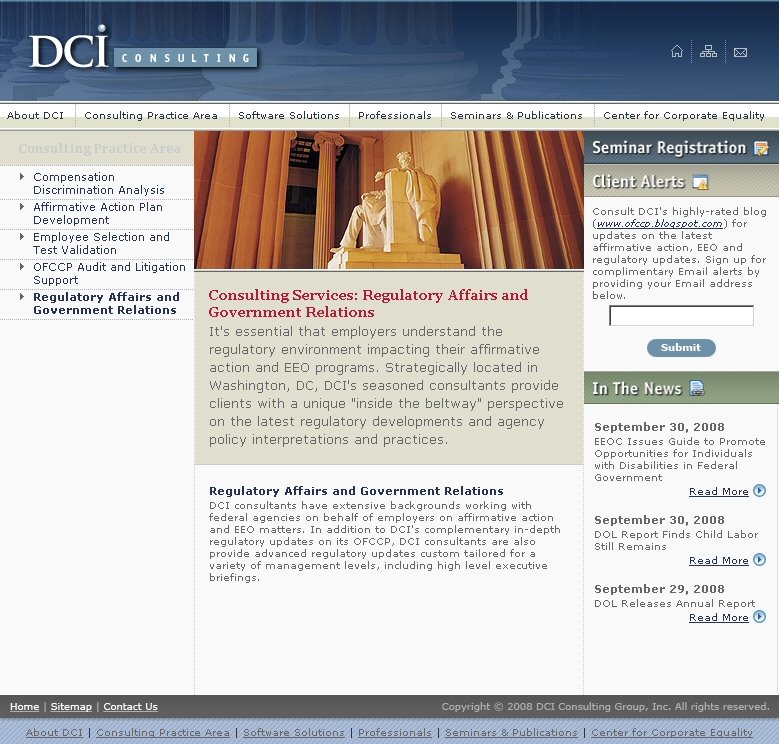This screenshot displays the homepage of the DCI Consulting website. The layout starts with a sophisticated header in blue, featuring an image hinting at the formal columns of a classical building, symbolizing stability and professionalism. The company name, "DCI Consulting," is prominently displayed in crisp white text within this header.

Below the header, the main navigation area is set against a tan background and includes the following menu options: About DCI, Consulting Practice Area, Software Solutions, Professionals, Seminars and Publications, and Center for Corporate Equality. These menu options are horizontally aligned, facilitating easy access to different sections of the website.

On the left side of the screenshot, a vertical navigation bar lists specific consulting practice areas. The sections here include titles such as Compensation Discrimination Analysis, Affirmative Action Plan Development, Employee Selection and Test Validation, and OFCCP Audit and Litigation Support. As you scroll down the navigation bar, there is a distinct section in bold black text labeled "Regulatory Affairs and Government Relations."

Towards the bottom of the screen, a horizontal menu provides essential links for site navigation, including Home, Sitemap, and Contact Us, running from left to right. All these elements together suggest a professional and comprehensive web presence aimed at providing detailed consulting services and resources.